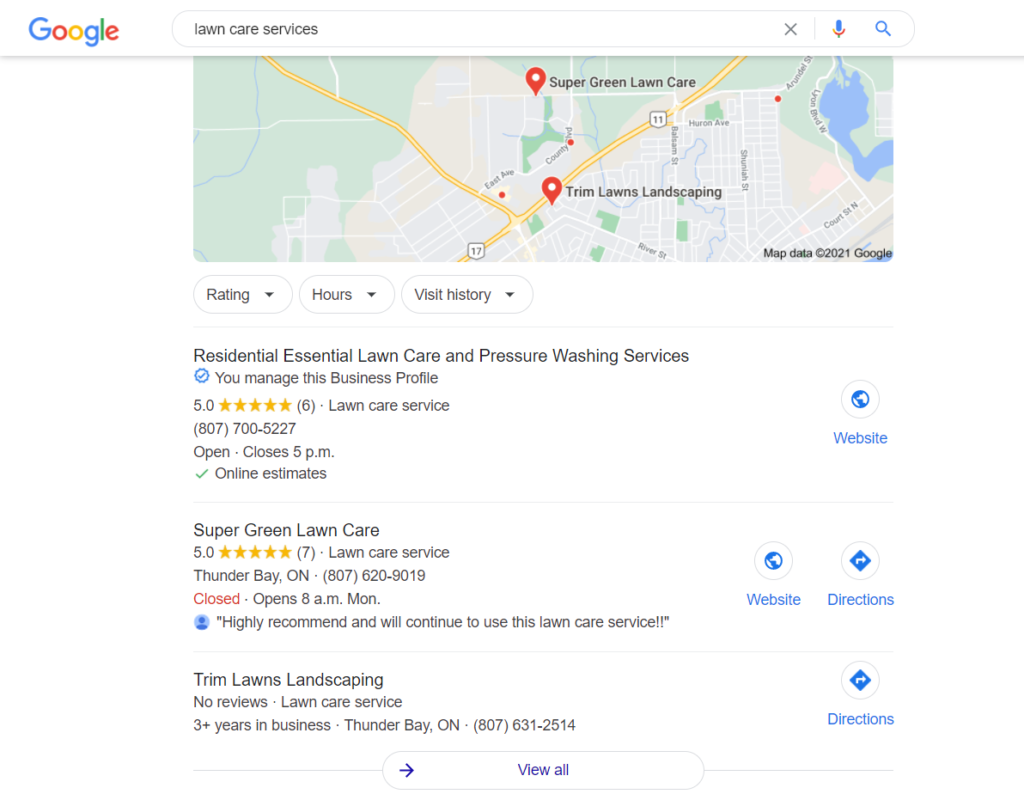In this screenshot of a Google search results page, the interface is prominently displayed with the familiar Google logo in its characteristic multicolored design situated at the top left corner. To the right of the logo, a search bar is visible, containing the query "lawn care services" alongside Google's microphone icon and a magnifying glass symbol, denoting search functionality.

Below the search bar is a partial view of a map rendered in light green, white, and blue hues, representing land, roads, and water bodies, respectively. Key roads, including highways 17 and 11, are illustrated in white and yellow. Two businesses are highlighted on the map: "Super Green Lawn Care" appears first, followed by "Trim Lawns Landscaping."

Under the map, there are three interactive buttons, labeled "Rating," "Hours," and "Visit History," each featuring a dropdown menu. The businesses listed below these buttons are, in order:
1. Residential Essential Lawn Care and Pressure Washing Services
2. Super Green Lawn Care
3. Trim Lawns Landscaping